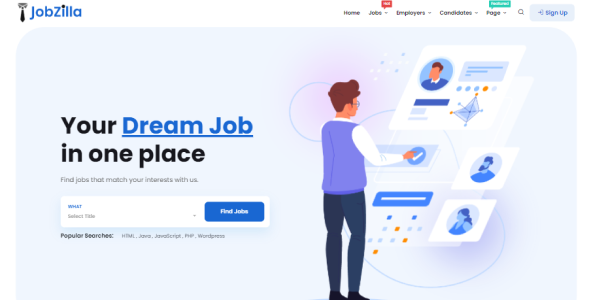In the top left corner, there is a symbol resembling a razor with a handle, possibly intended to be a stamp. To the right, the text "Jobzilla" appears in blue, circular, and somewhat bubbly font, with the dot on the 'i' colored black instead of blue. Further to the right, a menu bar is visible. The first menu option is "Home" in small black lettering, followed by "Jobs" which includes a small red blurb with white text that is indecipherable and an arrow indicating a drop-down menu. Next is "Employers", also linked to a drop-down menu. Following that is "C-A-N-D", with the full text unclear, and "Page", another drop-down menu option. Towards the far right of the menu is a light blue rectangle with the blue text "Sign Up".

Below the menu, a large banner with rounded edges occupies the main part of the website. On the left side of the banner, black text reads "Your Dream Job" with "Dream Job" underlined in blue and then continuing in black with "In One Place." Underneath, in gray text, it states "Find Jobs That Match Your Interest With Us." There is an input field configured as a drop-down menu with the prompt "What" in blue, bold lettering, and "Select State" in light gray lettering. Adjacent to this field is a rectangular button with rounded edges, a dark blue background, and white text reading "Find Jobs."

On the right side of the banner, a man is depicted wearing a light purple sweater vest and black slacks. He has short golden-brown hair and glasses, extending his right arm to interact with a touchscreen. Several windows are visible on the screen he is interacting with, one of which displays a cartoon-style user icon of himself.